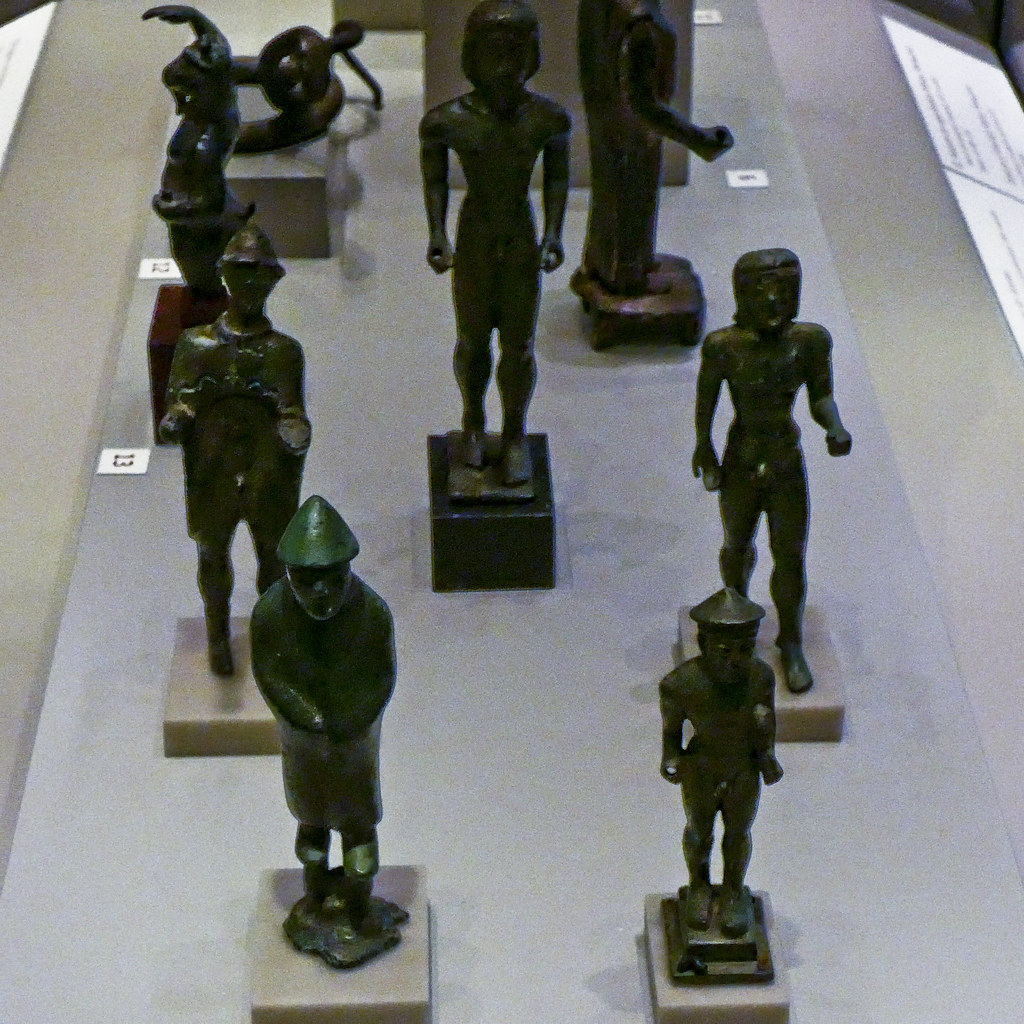This photograph appears to be taken inside a museum display case, showcasing a collection of dark green statues, likely made of pewter, positioned on a dark gray slab or table. The image quality is quite poor and grainy. The display is arranged in a structured manner, with statues each adorned with small white tags bearing black numbers, such as "12" and "13". The statues, standing between six to ten inches tall, predominantly face towards the camera or to the sides, although some are oriented more towards the center. 

In the bottom-left corner is a notable statue of a person with a triangular, cone-shaped hat and a beard, standing with arms crossed and two legs on a patch of dirt. Next to this figure, another statue stands on a pedestal, appearing to be naked and also wearing a triangular cap. This pattern continues with several other figures, some with arms separated from their bodies, giving them a more defined shape. The arrangement includes a mix of different poses and possibly roles, as some figures seem to represent farmers with conical hats, while others, with more pronounced helmets, might depict soldiers.